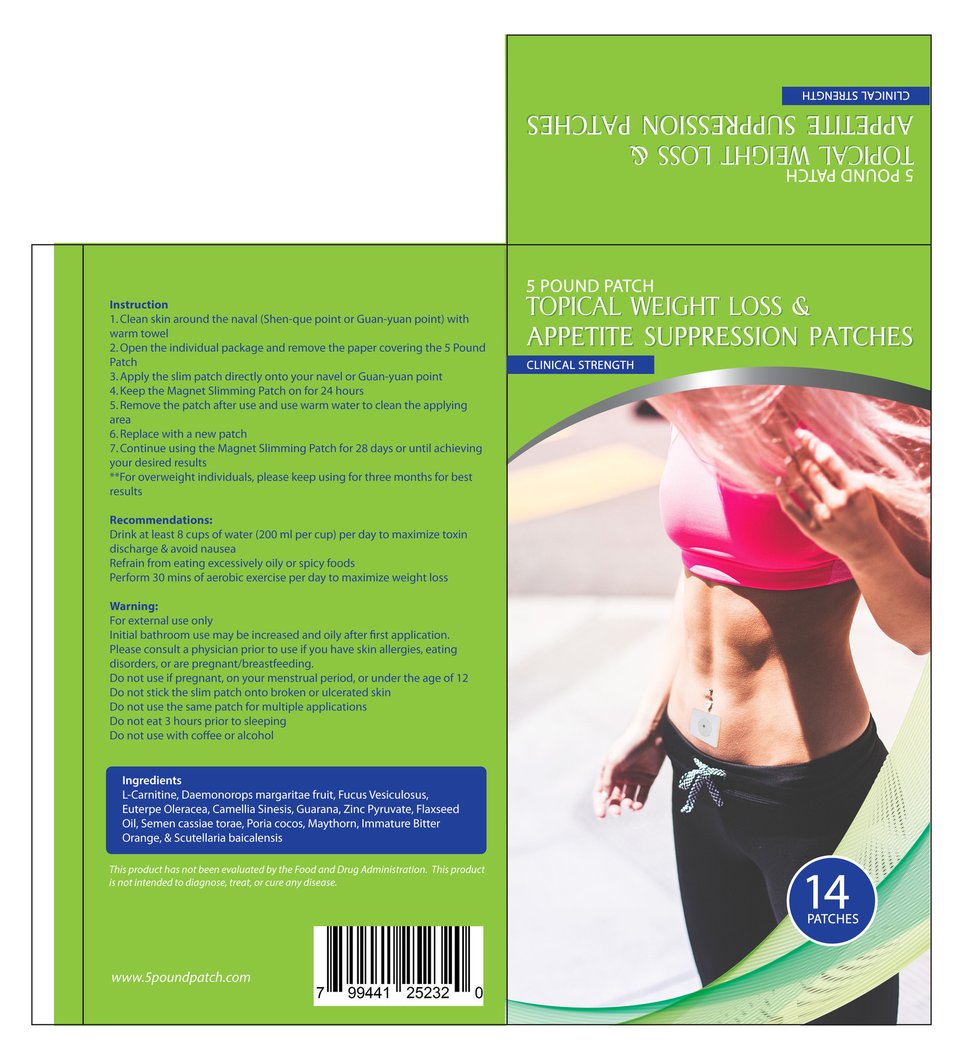The image depicts a flattened, opened cardboard box designed for a weight loss product known as the "5 Pound Patch." The main color scheme of the box is green with blue accents, featuring repeated text that highlights "topical weight loss and appetite suppression" and marks the product as "clinical strength." The central visual element is a fit woman with long blonde hair, wearing a pink sports bra and black pants that are tied with a white string. She has a visible patch just below her belly button. The front cover indicates that the box contains "14 patches" and prominently displays the website "5lbpatch.com." Additionally, detailed instructions and ingredients are listed on the side panel in blue text against the green background. Notable ingredients include L-carnitine and margarita fruit. A barcode is located at the lower left, reinforcing the product’s commercial presentation.